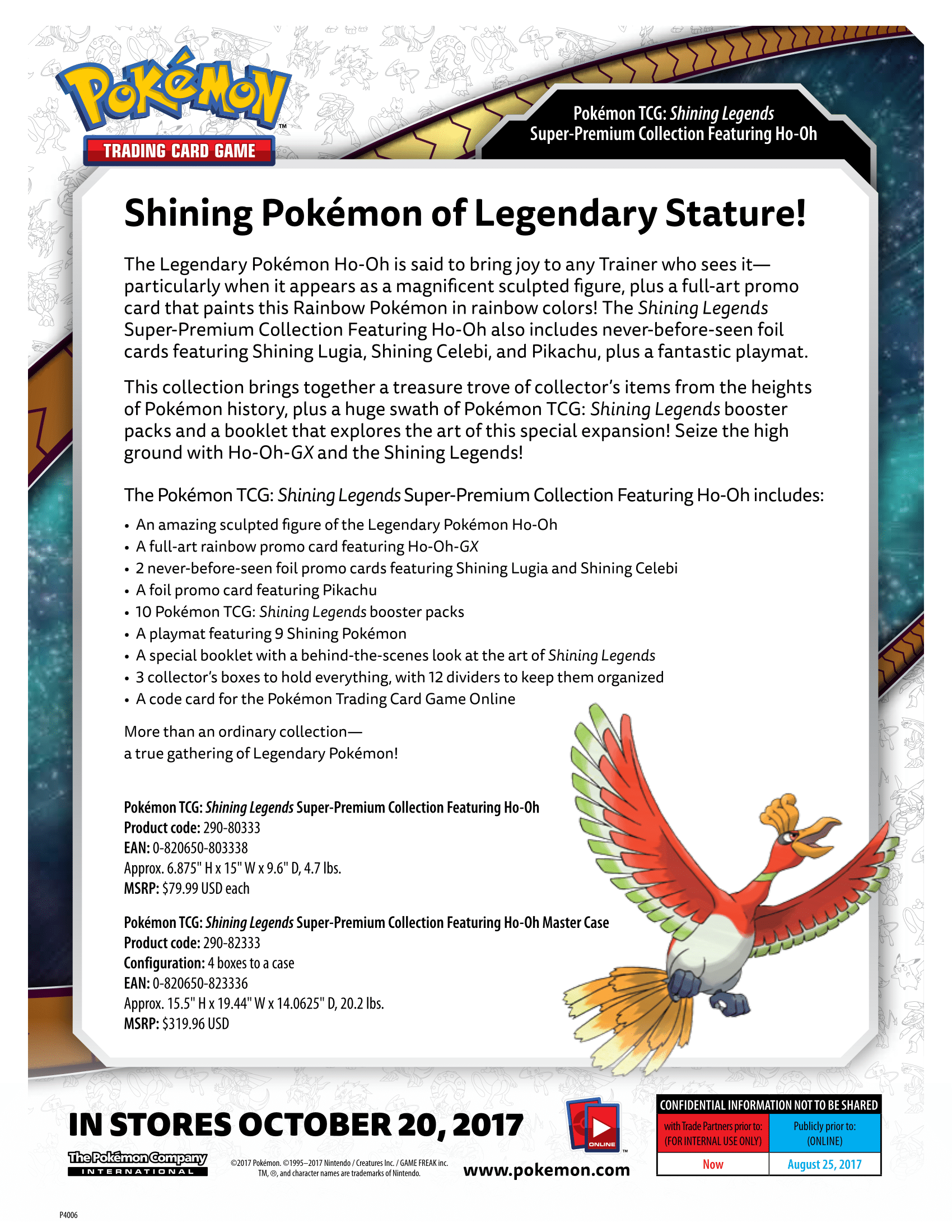### Pokemon TCG Shining Legends Super Premium Collection Featuring Ho-Oh

Experience the ultimate homage to Pokemon lore with the Pokemon Trading Card Game (TCG) Shining Legends Super Premium Collection, spotlighting the Legendary Pokemon Ho-Oh. This captivating assortment boasts a meticulously crafted Ho-Oh figure, designed to spark joy in any trainer's heart, as well as a vibrant, full-art promo card featuring Ho-Oh GX in stunning rainbow hues.

The collection also includes never-before-seen foil cards of Shining Lugia and Shining Celebi, and a foil card of the fan-favorite Pikachu. Enhance your battle strategies and add to your collection with ten Shining Legends booster packs. A special playmat showcasing nine Shining Pokemon and a behind-the-scenes art booklet elevate this collection from great to legendary.

To keep everything organized, the set provides three collector’s boxes with twelve dividers, making this not just a collection but a treasure trove of Pokemon history. Additionally, a code card for the Pokemon Trading Card Game Online ensures you can enjoy these exclusive items digitally as well.

#### What's Inside:
- A beautifully sculpted figure of the Legendary Pokemon Ho-Oh.
- A full-art, rainbow promo card featuring Ho-Oh GX.
- Two never-before-seen foil promo cards of Shining Lugia and Shining Celebi.
- A foil promo card of Pikachu.
- Ten Pokemon TCG Shining Legends booster packs.
- A playmat featuring nine Shining Pokemon.
- A booklet offering a behind-the-scenes look at the art of Shining Legends.
- Three collector’s boxes for storage with twelve dividers.
- A code card for the Pokemon Trading Card Game Online.

#### Product Specifications:
- **Product Code**: 290-80333
- **EAN**: 0820650-803338
- **Dimensions**: Approximately 6.875 inches (height), 15 inches (width), 9.6 inches (diameter)
- **Weight**: 4.7 pounds
- **Manufacturer Suggested Retail Price**: $79.99

#### Mastercase Details:
- **Product Code**: 290-82333
- **Configuration**: Four boxes per case
- **EAN**: 0820650-823336
- **Dimensions**: Approximately 15.5 inches (height), 19.44 inches (width), 14.0625 inches (diameter)
- **Weight**: 20.2 pounds
- **Manufacturer Suggested Retail Price**: $319.96

#### Release Information:
- **Available In Stores**: October 20th, 2017
- **Produced By**: Pokemon Company International
- **Confidentiality**: This information is confidential and intended for internal use only. 

For more information, visit [www.pokemon.com](http://www.pokemon.com).

### Trademarks:
- **Pokemon** © 1995-2017 Pokemon / Nintendo / Creatures Inc. / GAME FREAK inc. All rights reserved.

### Note:
This collection is a must-have for any Pokemon TCG enthusiast, offering a comprehensive and exquisite set of items, from exclusive promo cards to detailed collectibles. Don't miss the chance to add this legendary collection to your Pokemon TCG adventure.